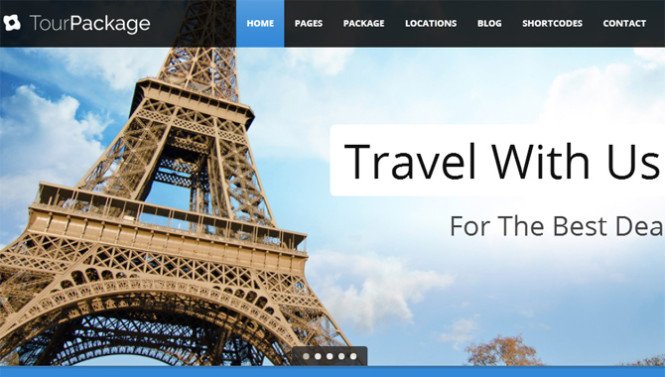This is a screenshot capturing the homepage of a travel website. At the top, a black bar spans the width of the screen, serving as the navigation bar. On the far left side of this bar, there is a four-petal flower-like logo symbol. Adjacent to it, the text reads "Tour Package" with "Tour" in gray and "Package" in white. 

The navigation bar features several white buttons; the first one, labeled "Home," is highlighted in blue, indicating the current page. The other navigation options include "Pages," "Package," "Locations," "Log," "Shortcodes," and "Contact," none of which are highlighted.

Below the navigation bar is a large image of the Eiffel Tower set against a blue sky filled with scattered clouds. Overlaid on this image is bold, black text proclaiming "Travel With Us." Positioned directly beneath this, in smaller text, it reads, "For the Best Deals," although the word "Deals" is partially cut off. At the bottom of the picture, a blue bar stretches across the screen, completing the visual layout of this part of the webpage.